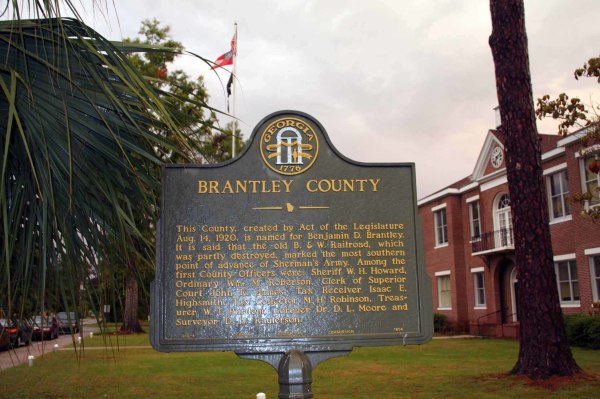The photograph captures a well-maintained lawn adorned with a historic plaque situated prominently in the foreground. The plaque is made of black iron with yellow text and features rounded top and rectangular bottom. At the top, the plaque prominently displays “Brantley County” and below it provides historical information, stating that the county was established by an act of the legislature on August 14, 1920, and is named after Benjamin D. Brantley. The text also notes that the old B&W Railroad marked the most southern advance of Sherman’s army, and lists the first county officers, although parts of the text are obscured by glare from the sun. Behind and to the right of the plaque stands a mature tree, and to the rear is a charming two-story brick building with a red roof. This building, adorned with a clock at the top of its gable, features a central balcony above an arched front door with steps leading up to it. Flanking the area are additional trees, and a flagpole with multiple flags can be seen waving in the background. To the left, vehicles are visible on a roadway or driveway, adding depth to the serene scene.